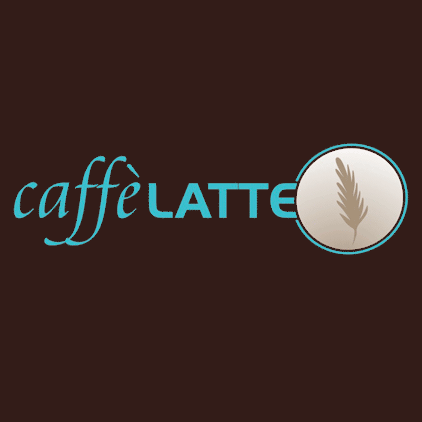This square image prominently showcases a company logo set against a very dark brown, deep mahogany background. Centrally placed, the logo features the brand name "CAFFE LATTE" written in light turquoise blue text. The word "CAFFE" is spelled in lowercase with two italicized, wavy 'f's, and an accented 'e', giving it a penmanship feel. Next to it, "LATTE" is in uppercase, designed with a thicker serif, more block-style font. Adjacent to "LATTE" is a circle with a thin turquoise outline. Inside this circle, there is a light tan, stylized feather, resembling cream art in a coffee, set against a white background.